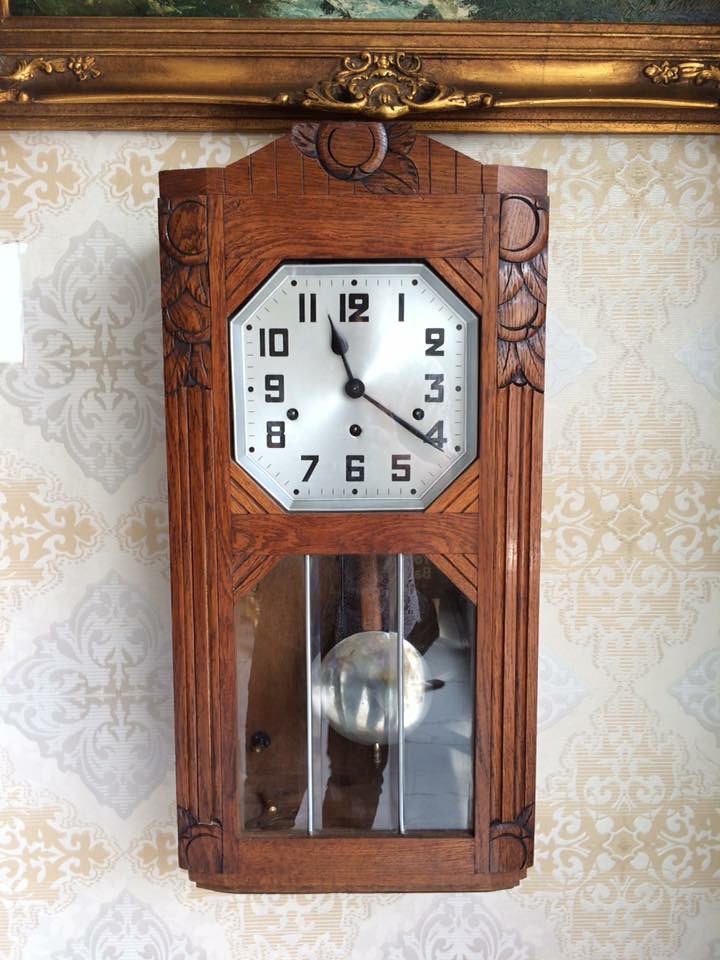This photograph showcases a richly detailed wooden wall clock hanging on a patterned wallpaper. The clock, carved from dark brown wood and shaped like a rectangle with a pointed top, features an octagonal white face adorned with black Arabic numerals and black hands. It reads 21 minutes past 11. The intricate design of the clock case includes a visible short pendulum through a lower window, hinting at the intricate mechanism within. To complement the scene, the ornate lower edge of a thick, gilt picture frame with elaborate designs peeks above the clock. The frame, golden in color, encases what appears to be an image with dark green and white elements, potentially floral. The wallpaper behind the clock is vibrant with gold and blue patterns, further enriching the setting.